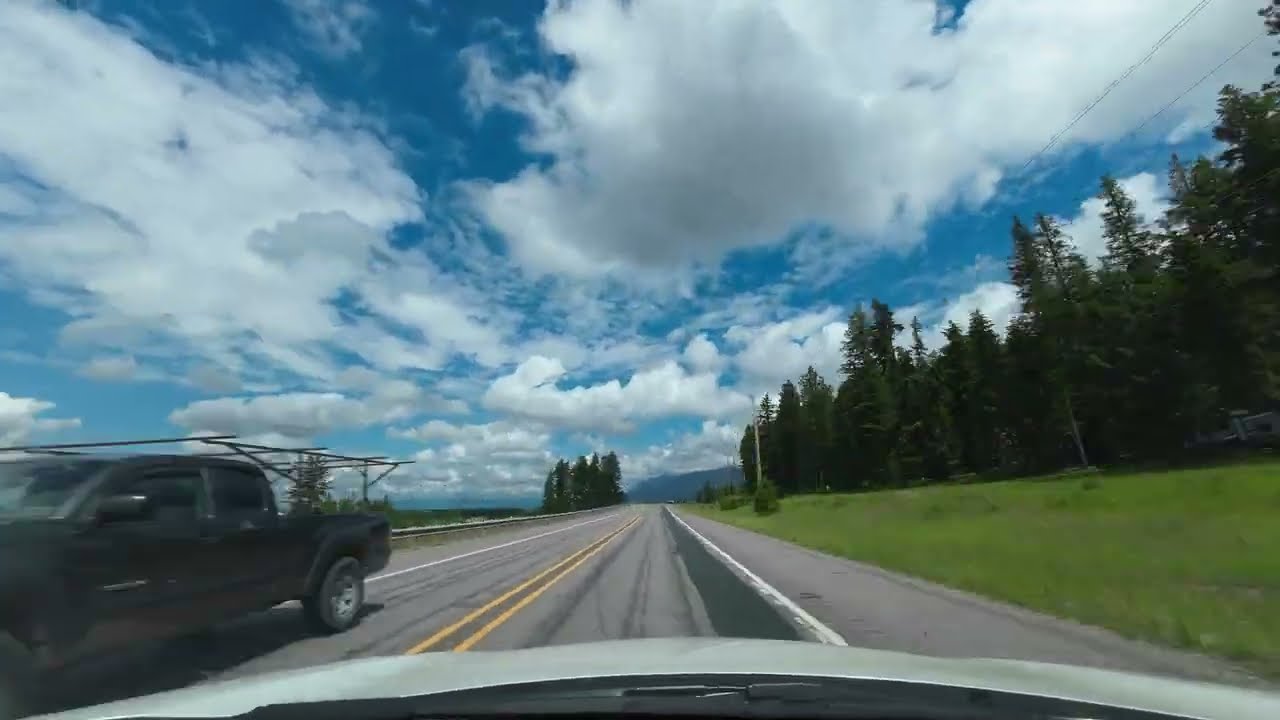This daytime photograph, captured from a dashcam within a white car, shows the vehicle's silver hood at the bottom of the frame. The car is driving along a gray road marked by two yellow lines down the center and white lines on either side. A black pickup truck with a steel frame at the back is partially visible in the opposite lane, just disappearing out of the image's bottom left corner. The road features a steel guardrail on the far left and a strip of grass to the right, leading to a line of mostly evergreen trees extending into the background. Power lines and a pole can be seen running alongside the right side of the street. Above, the sky is a deep blue with numerous white clouds, indicating a bright and sunny day. The general setting is a quiet, open road with no other vehicles, people, words, or numbers present.